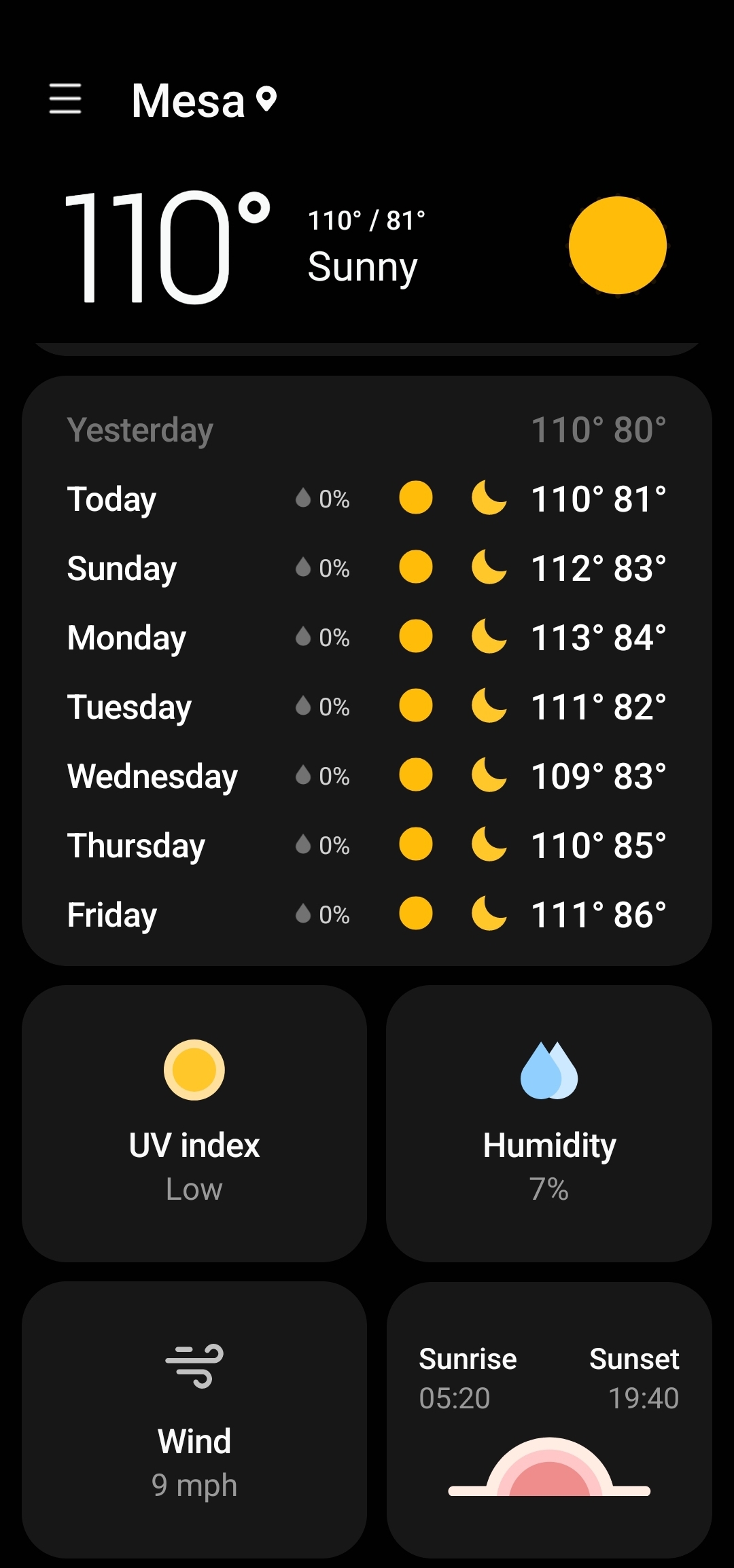The image showcases a detailed weather forecast interface against a black background, likely captured from a smartphone. In the top left corner, three small white horizontal lines are displayed beside the text "Mesa" with the current temperature prominently shown as "110 degrees" in white. Below this, more detailed weather information is provided with "110 degrees / 81 degrees, sunny." A bright yellow sun icon is situated on the right-hand side of this section.

On the left side, the word "yesterday" appears in gray, with corresponding temperatures "110 degrees / 80 degrees" listed beside it. Underneath, the day "today" is displayed in white, followed by a weather forecast for the week: "Sunday, Monday, Tuesday, Wednesday, Thursday, Friday." Everyday displays "0% chance rain," accompanied by symbols for a yellow sun and a yellow half-moon. The temperatures for the upcoming days are detailed as follows:
- Today: 110 degrees / 81 degrees
- Sunday: 112 degrees / 83 degrees
- Monday: 113 degrees / 84 degrees
- Tuesday: 111 degrees / 82 degrees
- Wednesday: 109 degrees / 83 degrees
- Thursday: 110 degrees / 85 degrees
- Friday: 111 degrees / 86 degrees

Below the weekly forecast are four smaller boxes arranged in two rows. The first box on the left features a yellow sun icon and the caption "UV Index low." To its right, a box labeled "Humidity" shows 7% with two raindrop icons. On the second row, the left box highlights "Wind" with a reading of 9 miles per hour, and the final box on the right indicates "Sunrise" at 05:20 and "Sunset" at 19:40.